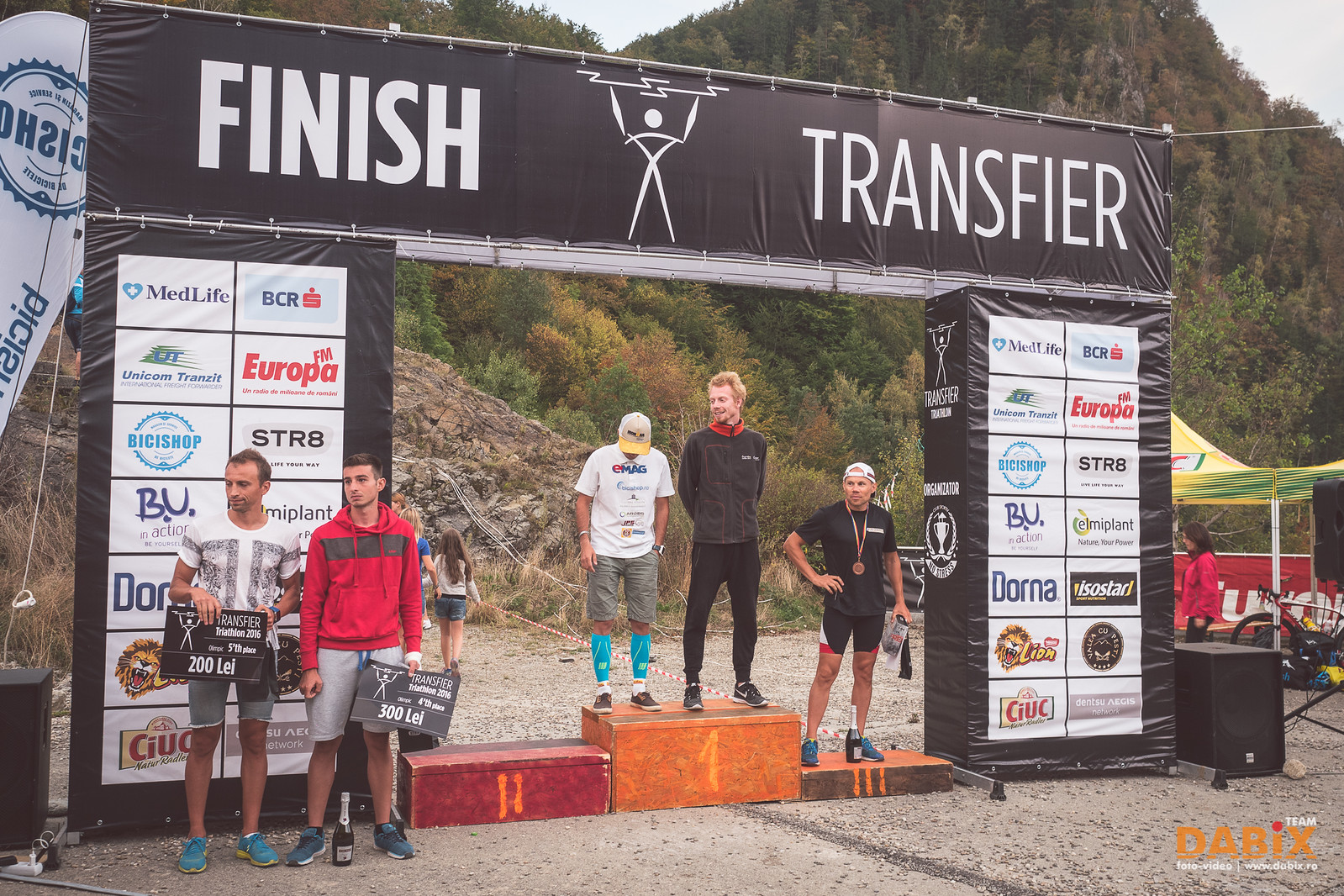In the photograph, a mid-afternoon outdoor award ceremony unfolds before a scenic backdrop of green-clad mountains and rocky hills. The centerpiece is a stage-like scaffolding structure adorned with black tarps displaying numerous sponsor logos, reminiscent of business cards, on both sides. At the top, bold white uppercase letters spell out "FINISH TRANSFIER" alongside a logo of a man with raised arms.

Three podiums are centrally placed, highlighting the first, second, and third place winners of what appears to be a race. The middle, tallest podium, marked with the number one, accommodates two men side by side, suggesting a tie for first place. The first man, wearing a white t-shirt, grey shorts, blue socks, and a white baseball cap with a yellow bill, looks downwards. Beside him stands a taller man in a grey, fully-zipped long-sleeve shirt, black pants, tennis shoes, and sporting short blonde hair. On the podium to the right, marked with a three, a man stands wearing a backwards baseball cap, a pendant, a short-sleeved black t-shirt, and black bicycle shorts.

Two additional men stand to the left in front of one of the black tarps, one dressed in a red hoodie and the other in a white shirt, both holding small black signs. The setting is vibrant, with clusters of greenery on the mountain peaks and a yellow pop-up tent to the right of the stage. A black speaker hints at impending announcements, completing the tableau of anticipation and achievement.